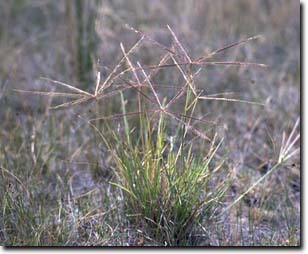This image, set against a pure white background with an artificial black shadow along the bottom and right side, captures a small, focused glimpse of natural scenery. Dominating the center of the frame is a tuft of grass with varied shades of dark green and light yellow, accentuated by light brown, helicopter-shaped seeds radiating outwards. The foreground features proud, sprouting green grasses, standing in stark contrast to the predominantly dead and brown surroundings. The background, increasingly blurred, showcases shorter, withered grass interspersed with small green patches. On the rear left, a taller plant with green and light brown hues adds depth to the scene. The overall effect highlights the resilience of new growth amidst a landscape largely characterized by dryness and decay.